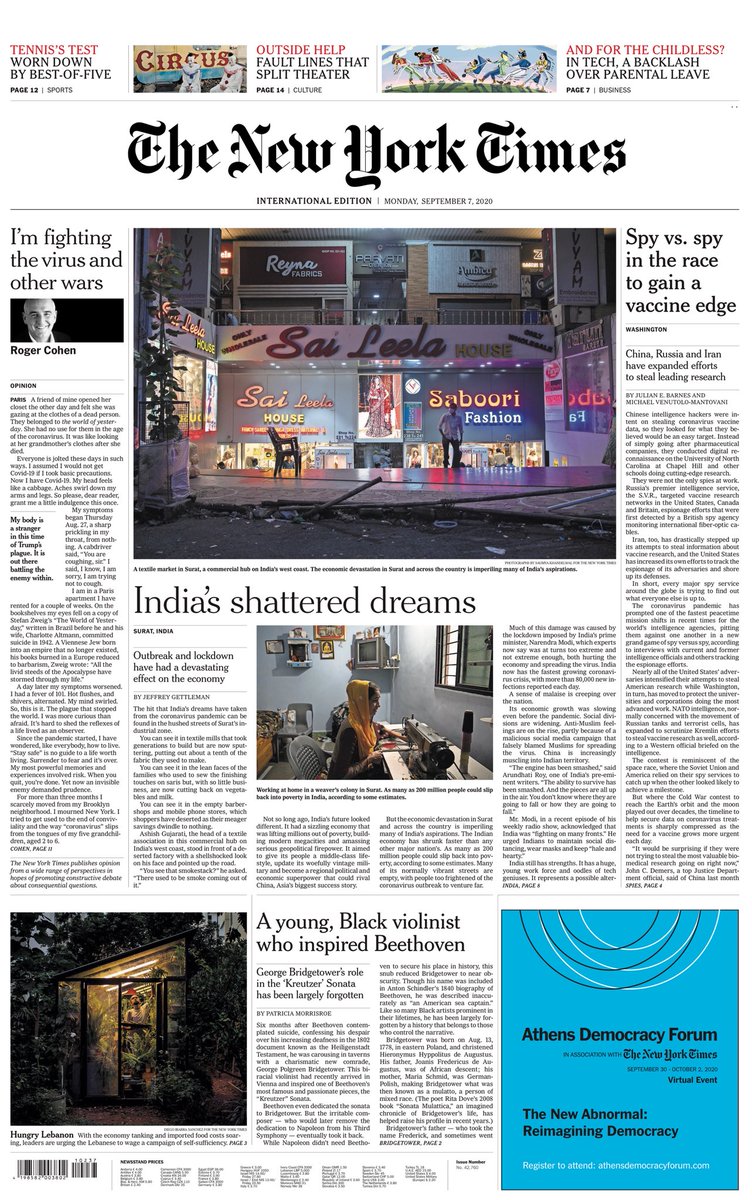Newspaper Front Page Analysis:

The front page layout of The New York Times International News dated Monday, September 7, 2020, features a variety of headlines and images against a predominantly white background, with black text at the top. The main headline reads, "World Tennis Test Worn Down by Best of 5," capturing attention with bold typography. Below this, another significant feature titled "Outsider Help or Fault Lines" discusses the fissures within a theater community, accompanied by an eerily depicted image of circus clowns.

Adjacent to these articles, a cartoonish graphic highlights a piece titled, "For the Children List and Tag: A Backlash Over Parental Leave," suggesting societal debates regarding parental rights. 

On the left-hand column, a headline reads, "I'm Fighting the Virus and Over the Wars," with a section characterized by a stark black background showcasing an older man named Roger Korn in a seemingly cluttered montage that makes it difficult to comprehend.

A vibrant image seemingly shot in a bustling Indian food market is featured prominently below these articles, referring to a story titled "Spy vs. Spy: The Race to Gain the Vaccine Badge," detailing the global competition to develop a COVID-19 vaccine. Another narrative titled "India Shattered Dreams" features a poignant image of a woman working at a sewing machine.

On the bottom left, an article titled "Young Black Woman by Witness Who Inspired Beethoven" is illustrated by a picture of a greenhouse. Adjacent to it, an advertisement with a blue background and black text highlights the Athens Democracy Forum, themed "The New Abnormal: Reimagining Democracy."

The front page is a rich tapestry of global issues, societal debates, and human interest stories, offering readers a deep dive into current events and emerging narratives.